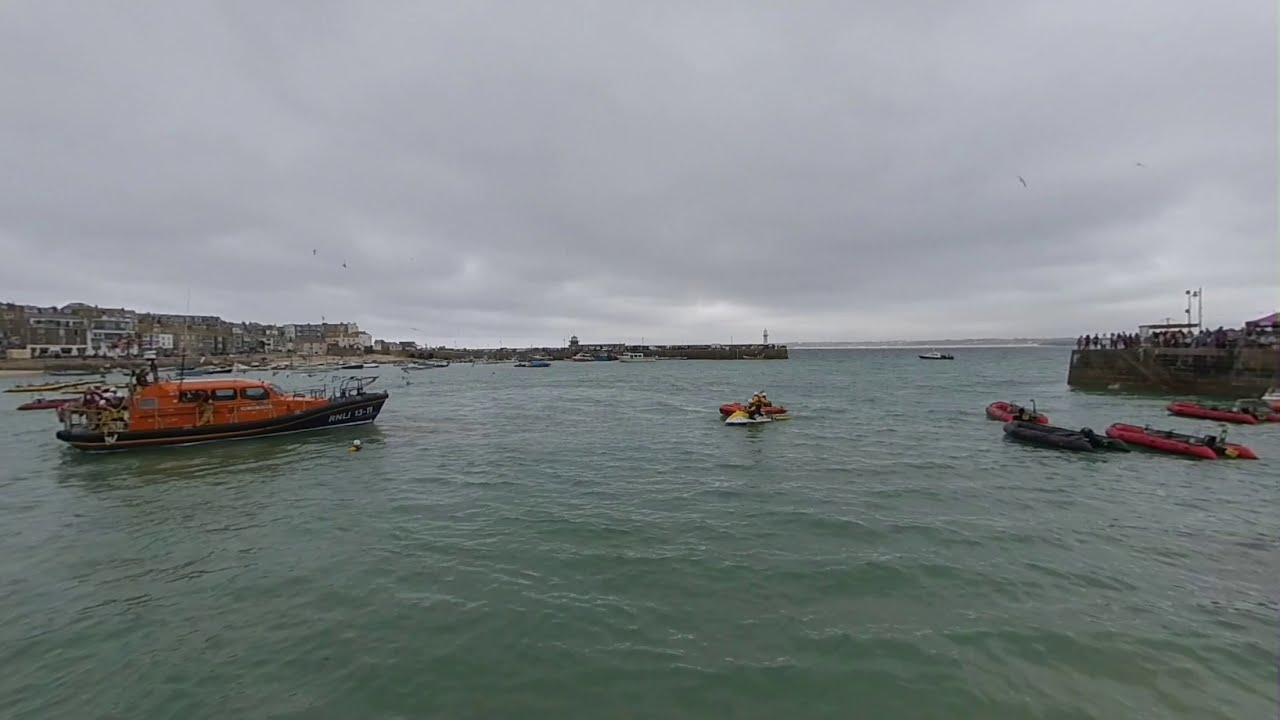The image depicts a lively harbor scene during daytime, featuring a vibrant array of boats and bustling human activity. The body of water is a greenish-blue, with its almost wave-less surface extending from the bottom to just above the middle of the image. Dominating the left side of the water is a large cruiser-type boat with an orange body and black hull, marked with "ANLI 13N," and crowded with people and equipment. A town stretches along the left horizon, characterized by multiple buildings, presumably residential, showcasing various colors like white, brown, and gray.

Just beyond the cruiser, towards the center, a yellow and white jet ski and a red boat move in the opposite direction of the cruiser. These are accompanied by other small vessels, including several unoccupied red and black inflatable rafts scattered across the water.

In the background to the right, a prominent stone pier teems with spectators, hinting at a communal gathering. Above, the sky is heavily overcast, dominated by gray and white clouds, which blanket the scene in a diffused, gentle light. The overall atmosphere captures a dynamic interaction between human activity and the natural and built environments of the harbor.